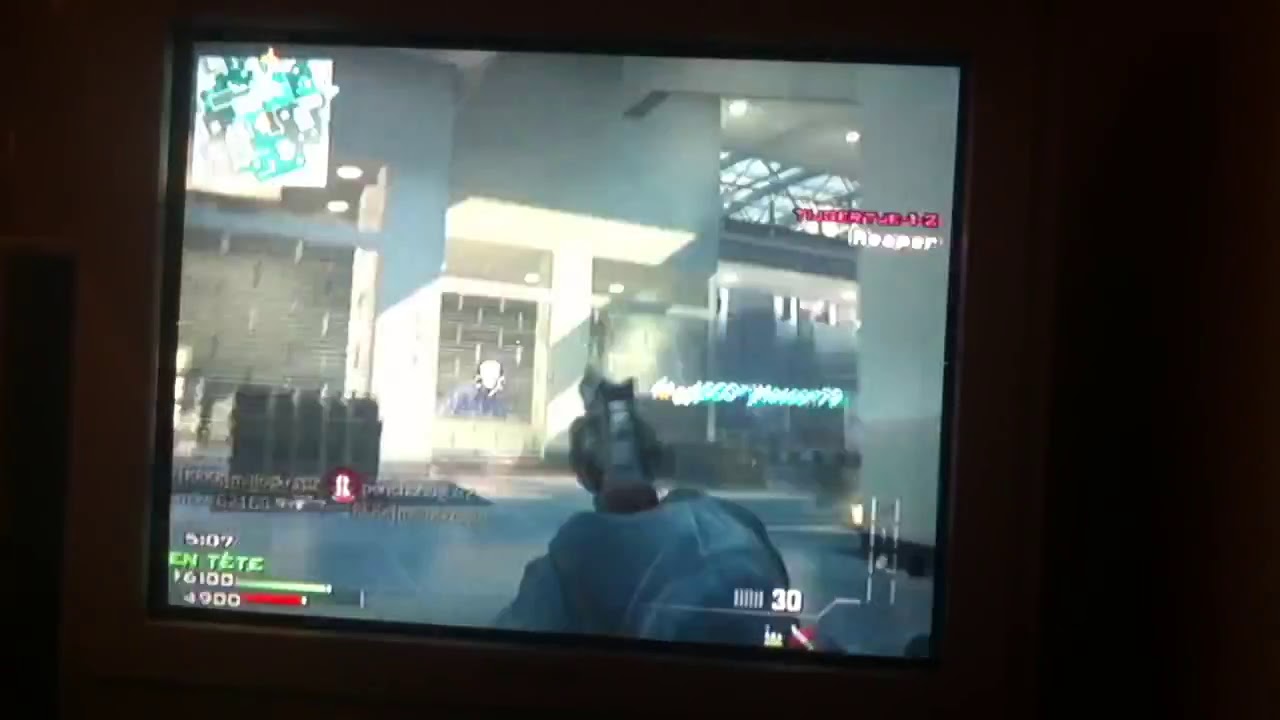The image is a slightly tilted, blurry, color screenshot from a first-person shooter video game, captured from a TV monitor set against a dark, dimly lit room. The central focus of the image is the monitor displaying a player's view of their hands, clad in black gloves, holding a pistol. The virtual environment appears to be the interior of a modern, white building with various objects and possibly mailboxes in the background. HUD elements are visible: a health bar and a shield bar on the bottom left, an ammo count with the number 30 and a knife icon on the bottom right, and a radar map on the top left. Red and white text, likely indicating an objective but unreadable due to the blur, is situated in the top right. The overall atmosphere is immersive, largely illuminated by the monitor itself, highlighting the intense gameplay experience.